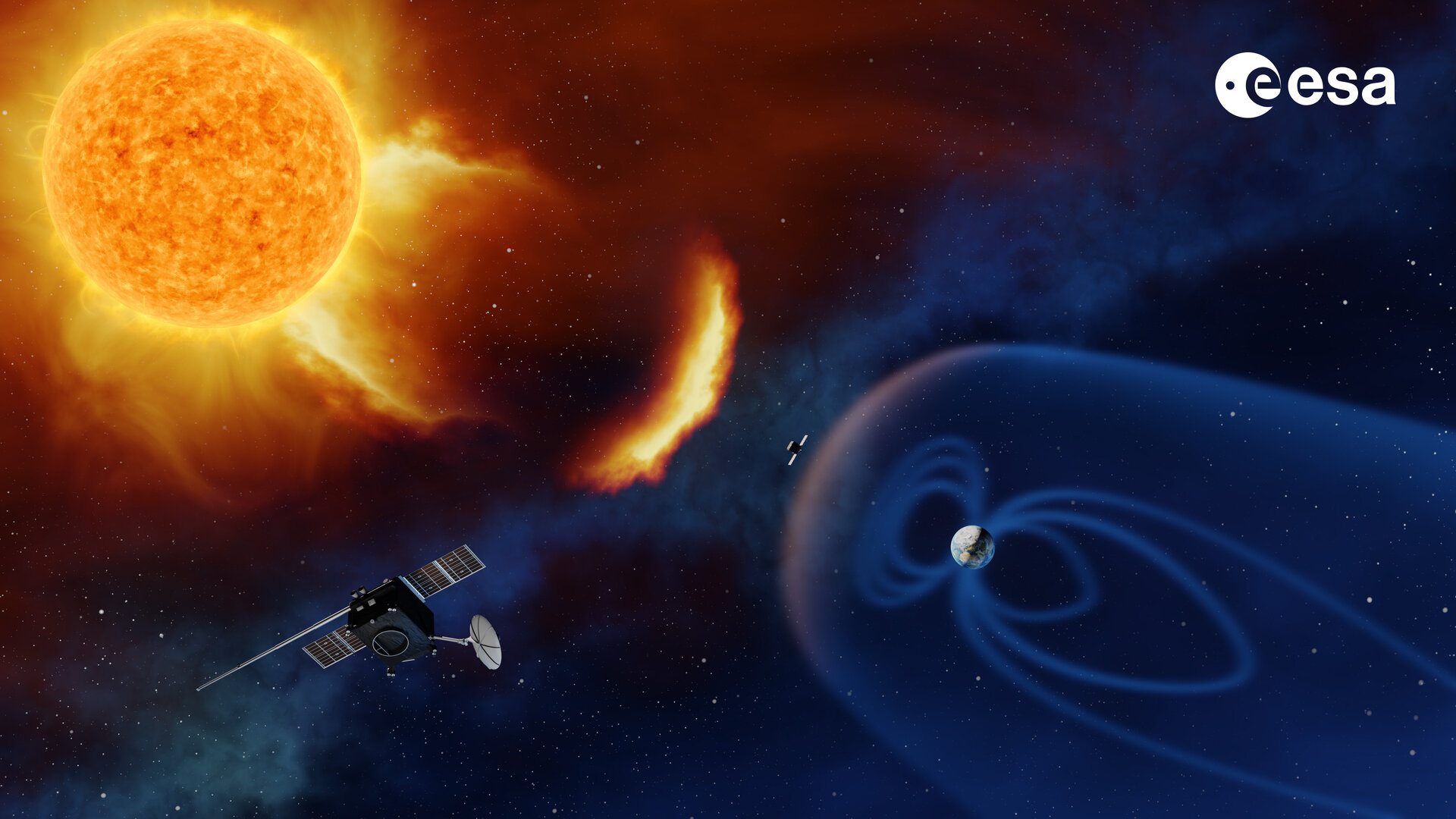In this image of outer space, the top left corner prominently features the Sun, depicted as a bright yellow and orange sphere radiating intense light and emitting fiery flares and a red aura into the dark blue expanse. To the right of the Sun, a small spacecraft or satellite is visible, appearing to float between the Sun and a tiny portrayal of Earth. The Earth is enclosed in a dark blue bubble-like aura. In the bottom left corner, we can see another black satellite with silver dishes. The top right corner of the image includes the logo "ESA" in white letters, indicating the organization responsible for the depiction. The entire scene is set against the backdrop of the dark, infinite void of space.